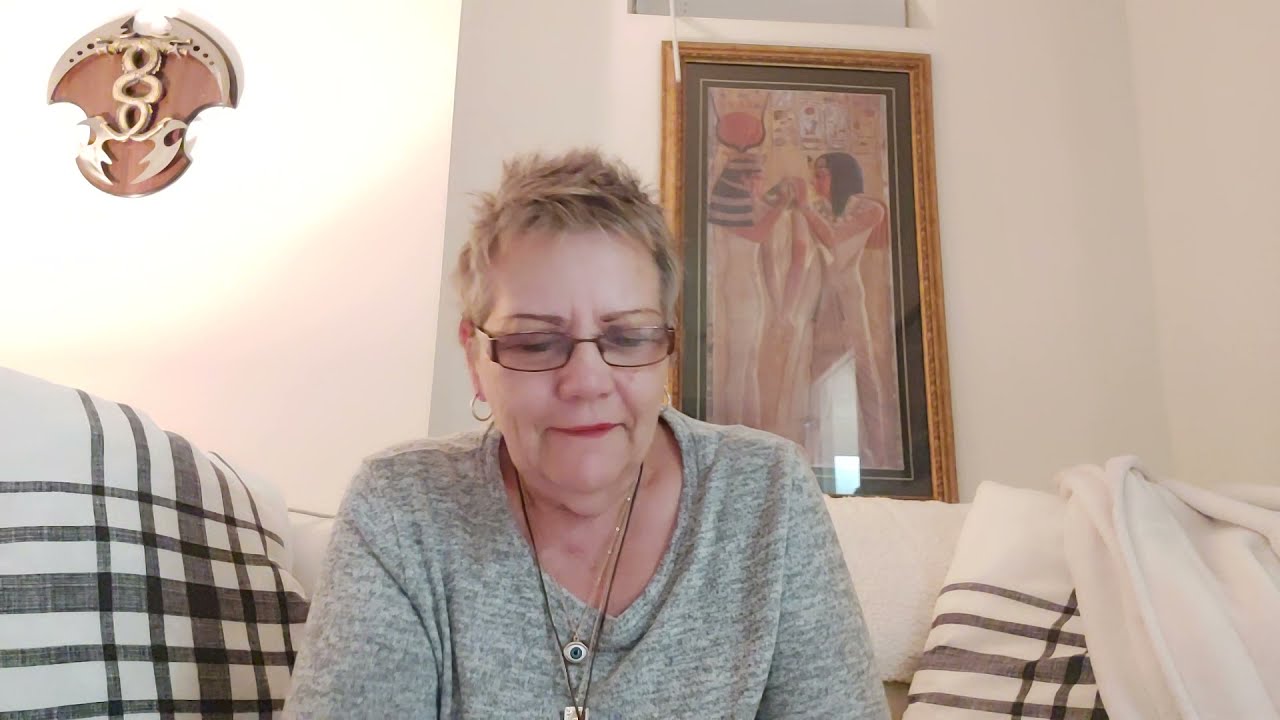The photograph captures an elderly white woman with short, spiky gray hair, wearing rectangular prescription glasses and small hoop earrings. She is seated on a beige couch adorned with beige and gray checkered pillows, and a white throw rug drapes over the right corner of the photo. The woman, dressed in a heathered gray long-sleeve shirt, is slightly leaning forward and looking down as if in mid-conversation. Around her neck, she wears multiple necklaces, including one with a distinct eyeball pendant and others with Egyptian-looking designs. The background features a wall with a glowing light source in the upper left-hand corner. Mounted on the wall are two prominent art pieces: a tall depiction of ancient Egyptian figures, possibly Cleopatra and Mark Antony, in a bronze-colored frame with a darker brown insert, and a wooden and brass plaque depicting intertwined snakes with blades.